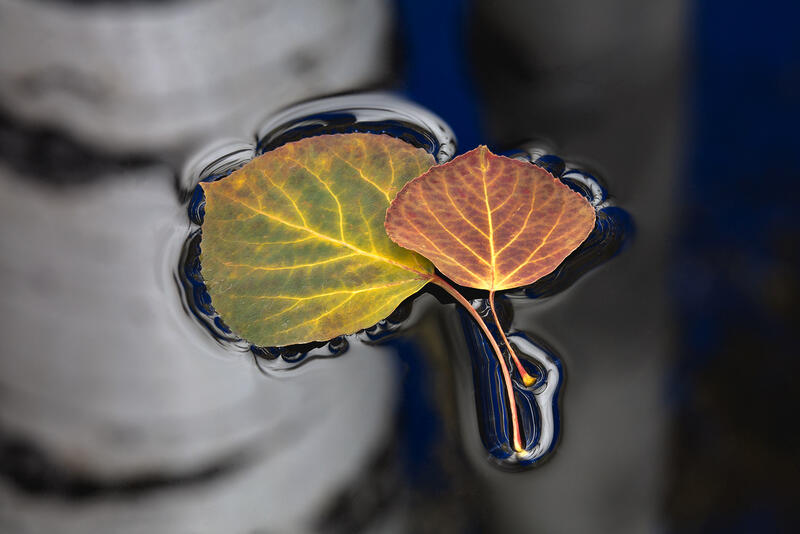In this detailed photograph, two leaves from the same type of plant float gently on the still, dark surface of water, which appears black due to its reflective nature. The larger leaf, positioned on the left, is primarily green with brownish-red edges, and it is threaded with a yellow vein system. Contrastingly, the smaller leaf on the right is a vivid red, adorned with yellow veins and a yellow stem. Both leaves are held afloat by the water's surface tension, creating visible indentations in the water that subtly enhance their depiction. The backdrop features a blurred reflection resembling an aspen tree with banded black and white markings, adding depth to the serene composition. The overall image seems enhanced, likely with filters, to accentuate the intricate interaction between the leaves and the water.